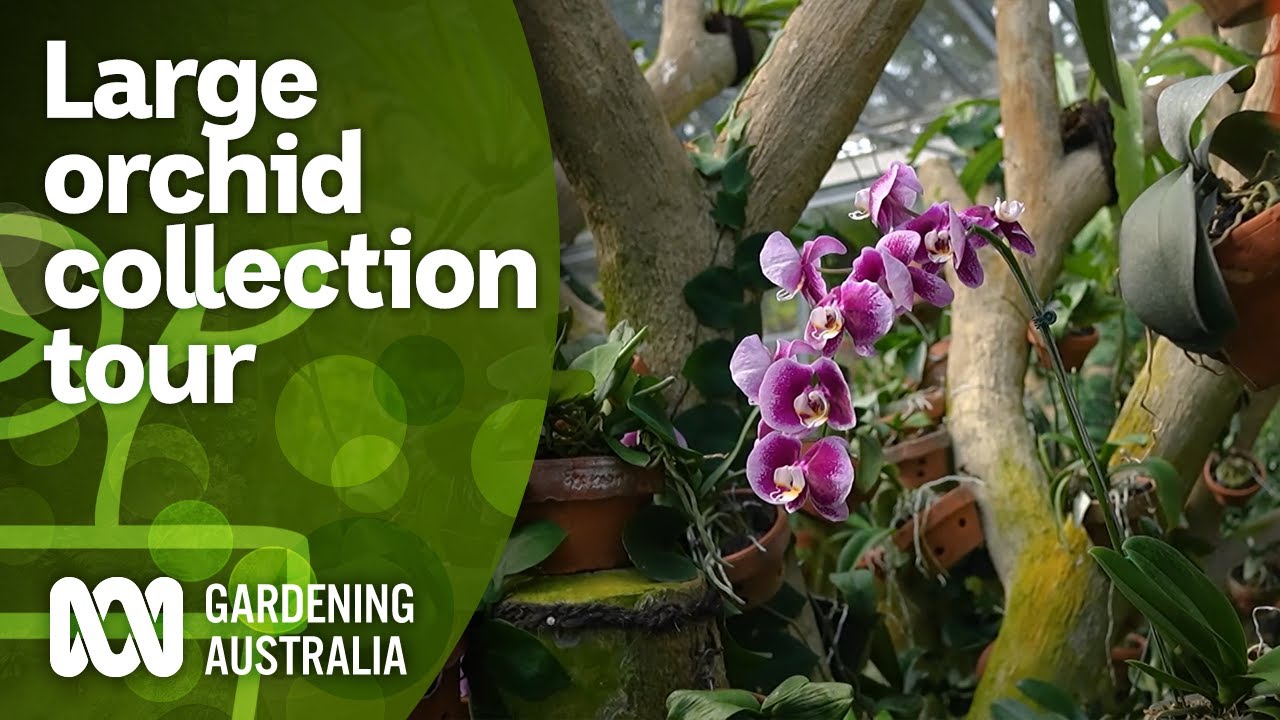The image depicts a vibrant and detailed infographic that could easily serve as a banner for a tourist or organizational website. On the right-hand side, the photograph showcases an inviting greenhouse filled with various plants, including a mix of lush trees in the foreground. A focal point within this greenhouse scene is a stunning potted orchid plant, boasting flowers with large, dark purple petals that fade to white at the edges. The flowers present a prominent structure, featuring a white and yellow center that adds to their unique appearance. The left-hand side of the image is dominated by a hunter green graphic background, which includes an illustrated plant icon. This portion of the infographic features white text that reads, "Large Orchid Collection Tour," with a logo resembling a swirly tube or a sideways spring at the bottom, which states, "Gardening Australia." The combination of these elements creates an eye-catching and informative visual advertisement for what appears to be a tour highlighting a diverse and extensive orchid collection.